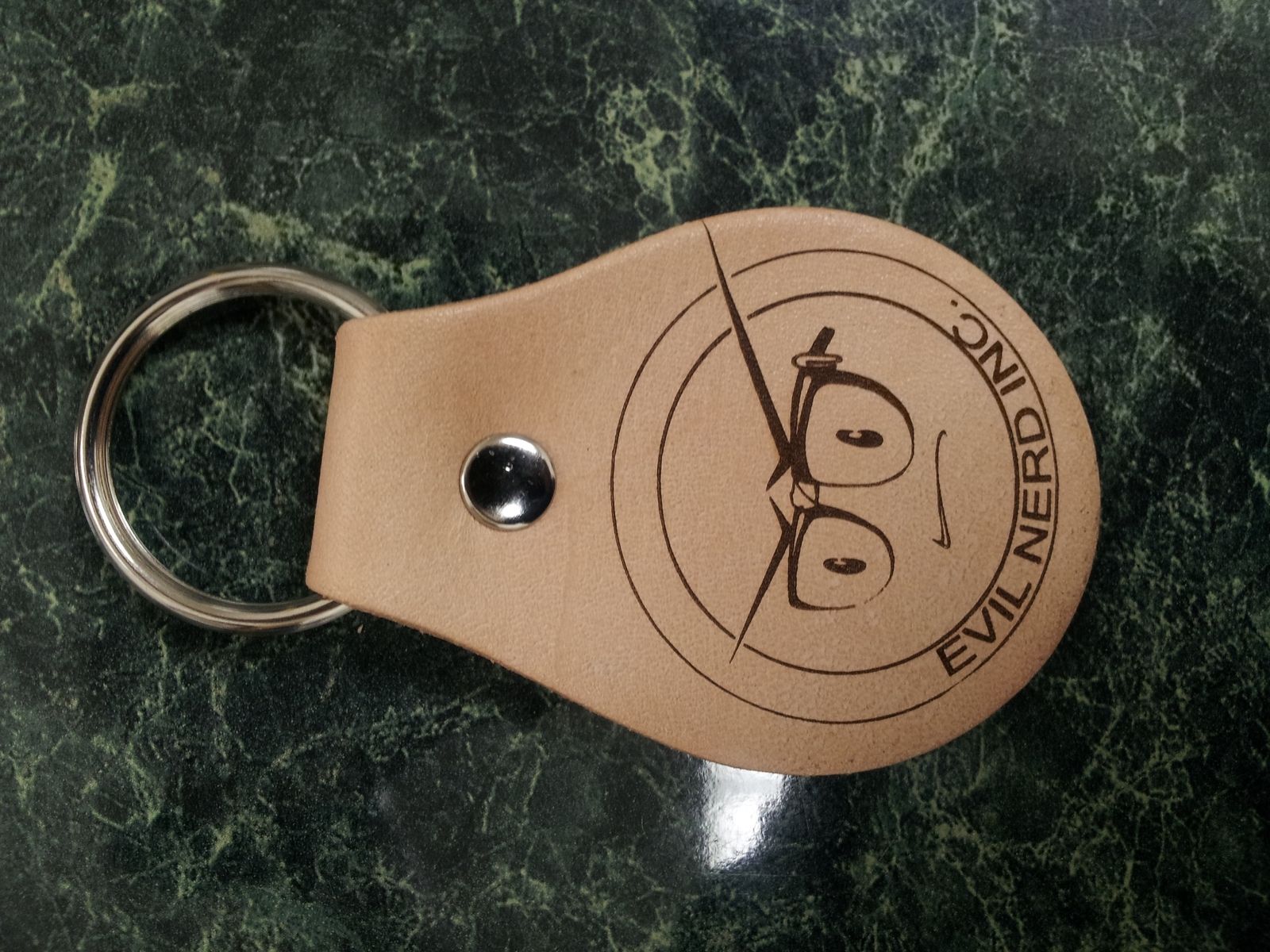This top-down photograph captures a brown leather keychain lying sideways on a dark green marble countertop, which features lighter green striations. The keychain, shaped similar to a squared-off teardrop, is attached to a silver key ring. Emblazoned on the front of the leather tab is a circular design with the text "Evil Nerd Ink" encircling a comical face. This face, appearing to make a mean expression, includes thick glasses, black dots representing eyes, and long, downward-pointing eyebrows—one eyebrow extending prominently to the edge of the keychain. Additionally, a small black line depicts a mouth, adding to the character's disgruntled look. The reflection of a light source and possibly the photographer's phone are also visible on the countertop.